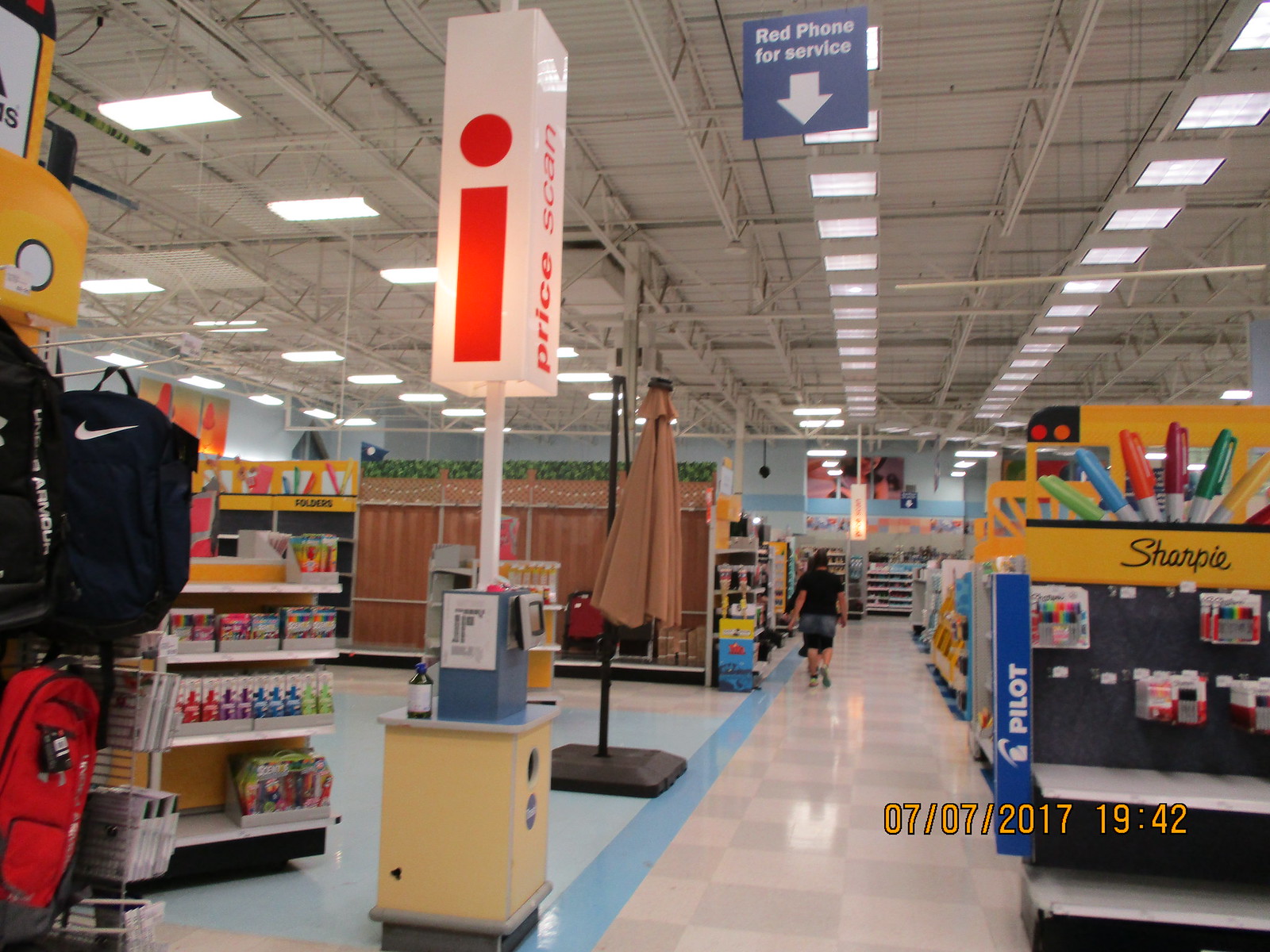This photograph captures the interior of a store, focusing down an aisle to the left. Dominating the view is a small desk area equipped with a price scanner, mounted on it. Above the desk, a white pole supports a large white sign featuring a red eye on one side and the words "Price Scan" on the other side. The store's ceiling is white with rows of lights illuminating the scene, and a blue sign hangs from the ceiling that reads "Red Phone for Service" with an arrow pointing downward.

On the right-hand side, there's a vibrant display for Sharpie markers, creatively designed to resemble a yellow school bus, with various Sharpies showcased below it. Towards the left side of the aisle, brightly colored shelves suggest an assortment of school supplies. A woman, dressed in either a denim skirt or shorts and a black t-shirt, walks away down the aisle, adding a dynamic human element to the scene.